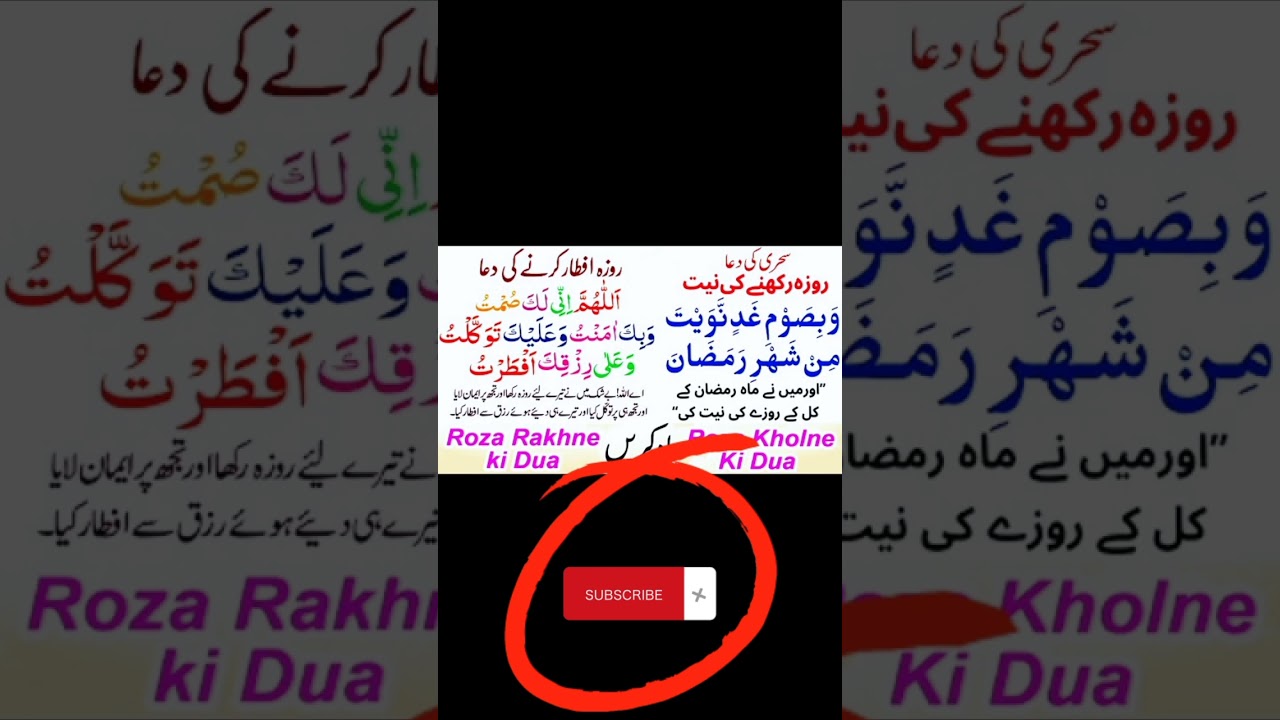The image depicts a complex digital interface featuring Middle Eastern script. The background consists of various colored scripts over a white backdrop. Dominating the bottom left and right corners are larger words in bright purple. Centrally, a black-bordered section contains a smaller version of the same image. Below this section, there is a prominent red button labeled "Subscribe," marked with a white X to the right and encircled dramatically in red, likely drawn using the paint feature. This button suggests a call to action for the viewer to subscribe. The overall composition is not in English, Chinese, or Russian, and appears to be in some form of Arabic writing, characterized by its distinct vowel markings. On either side of the central black banner, the script continues on a white background. The setup of the interface somewhat implies functionality seen in messaging systems, although no specific user names or messages can be identified.